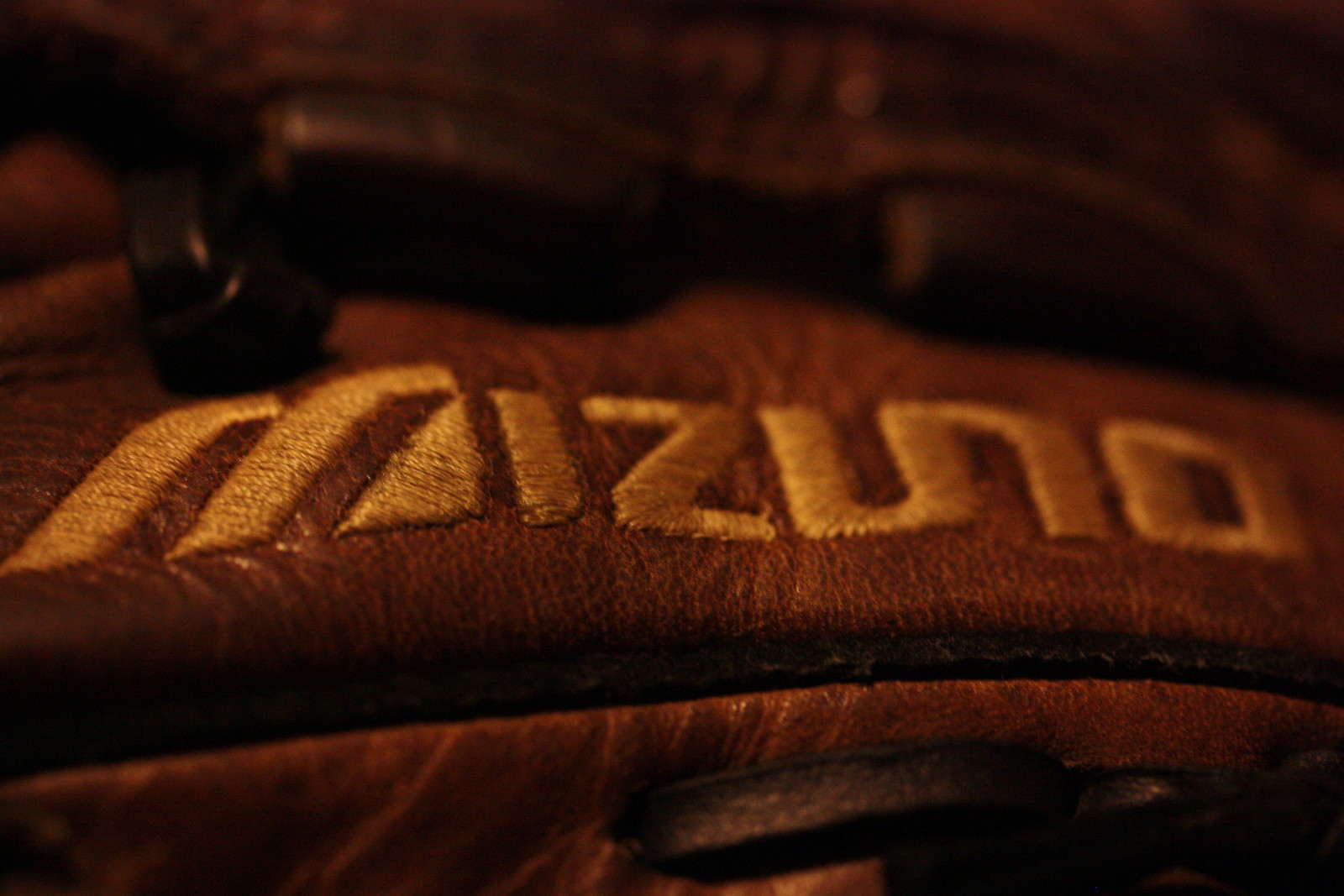The image is a detailed, close-up photograph of a Mizuno baseball glove, specifically a catcher's mitt. The glove is made of fine-grained, darker brown leather with multiple textures and shades, including soft, cushiony sections and dark brown borders. The Mizuno logo is prominently embroidered in yellow thread across the glove. The intricate craftsmanship is highlighted by both black and brown leather stitching and accents. In the background, there's a hint of a dark brown, possibly plastic latch, resembling a seat belt mechanism. The overall background remains muted, keeping the focus on the detailed textures and elements of the high-quality catcher's glove.